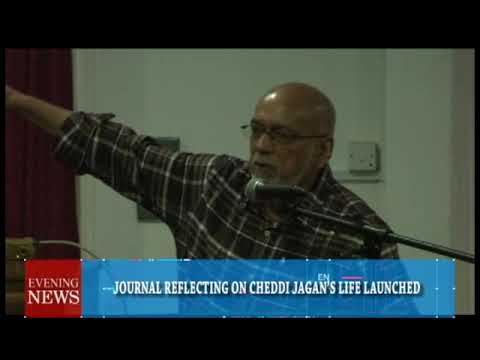In the image, a man with a shaved head, a gray beard, and a goatee is captured speaking into a black microphone, which is mounted on a stand. He is pointing to his right and seems to be in mid-speech. He is wearing glasses and a long-sleeve, black and white checkered plaid shirt. The background features a white wall with a visible outlet or box, and to the right, a maroon curtain and a door with a red hue. The lower part of the image displays an overlay with red text reading "Evening News" and a blue rectangle beneath it with white text that says, "Journal Reflecting on Cheddy Jagan's Life Launched," with 'Cheddy Jagan' spelled C-H-E-D-D-I J-A-G-A-N in a white Serif font. The man has a darker complexion and a shine on his bald head, suggesting the lighting is strong. The image, likely a still from a news program, provides a clear and detailed view of the subject and the setting, indicative of a formal or commemorative event.